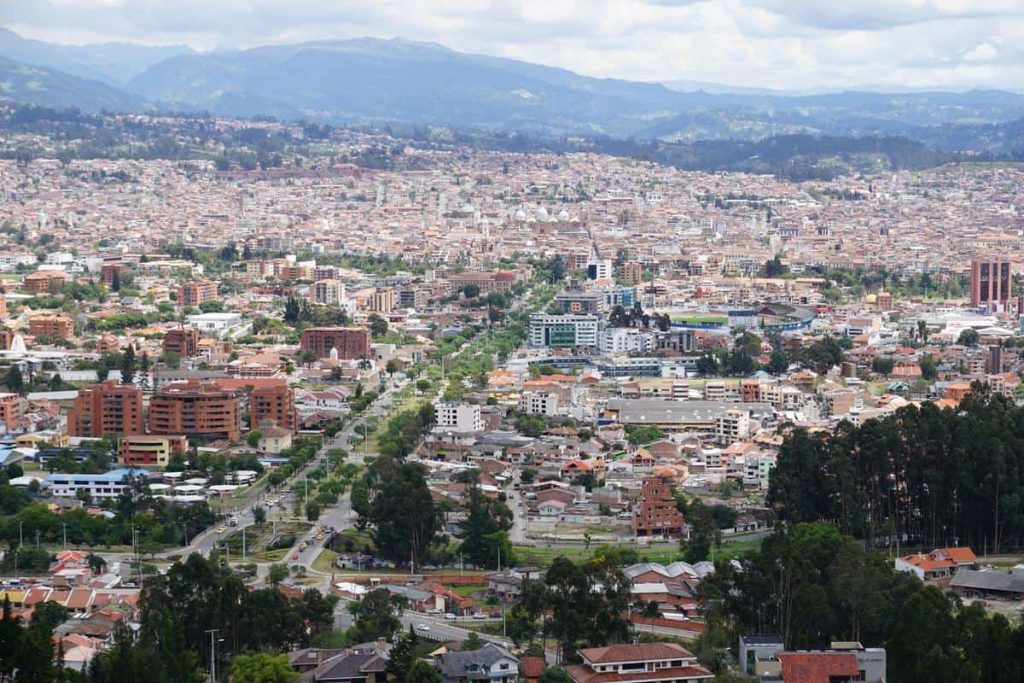This photograph offers a sweeping aerial view from a vantage point atop a high mountain, overlooking a sprawling suburban area near a city. The scene captures a blend of urban and suburban landscape, devoid of skyscrapers but featuring some prominent buildings. A main thoroughfare cuts diagonally from the bottom left to the top right, flanked by tree-lined strips of grass and dotted with a mixture of high-rise and smaller residential buildings, primarily in white and terracotta hues. Green spaces intersperse the foreground, transitioning into denser clusters of buildings toward the center of the image. Notably, churches and mosques are discernible in the distant mix. Mountains frame the backdrop, under a mostly cloudy sky, with occasional sunlight illuminating parts of the cityscape and roadways, adding a dynamic touch to the serene, partly cloudy day.